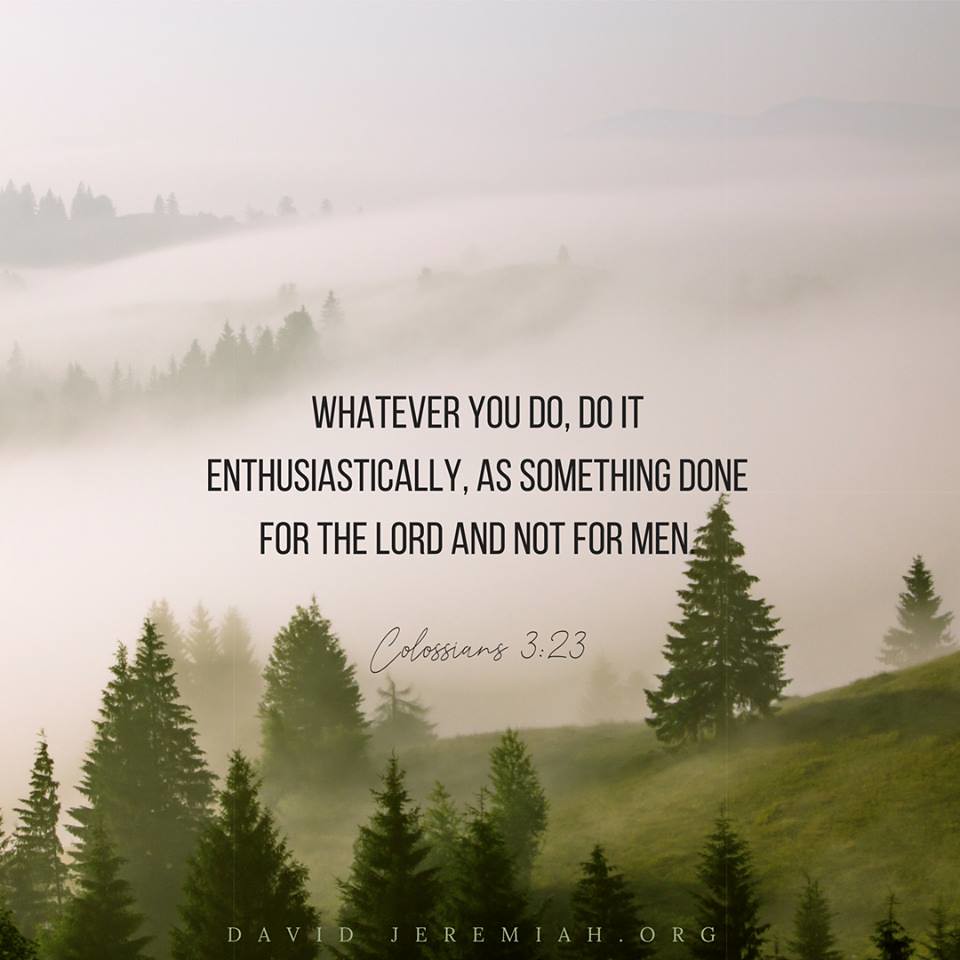The image is an artistic depiction of foggy, pine-covered hillsides. The composition features a slanted green hillside at the bottom, adorned with tall pine trees, mostly concentrated in the lower left corner. As your gaze ascends, the hillside is enveloped in thick, gray fog, creating a mystical atmosphere where more trees can be faintly seen fading into the mist. The top part of the image is light, almost ethereal, intensifying the foggy ambiance. Centered in the image is a motivational quote in black script: "Whatever you do, do it enthusiastically, as something done for the Lord and not for men." Beneath this, the verse reference "Colossians 3:23" is elegantly written in cursive. At the very bottom, in white text, is the web address "DavidJeremiah.org." This image has no border, focusing all attention on the serene and spiritual scene.